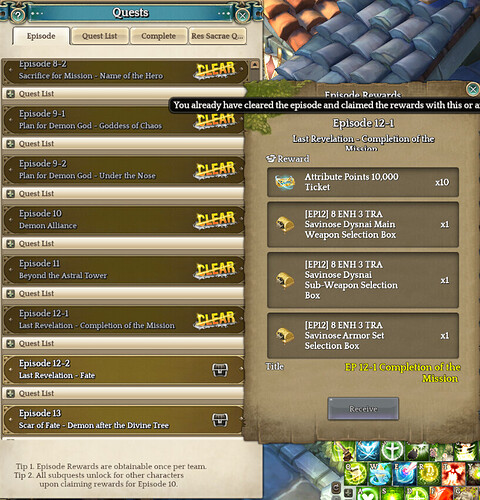This image is a detailed screenshot likely taken from a computer or mobile device, illustrating a game interface. The interface is dominated by a central screen filled with vivid colors such as blue, white, various shades of brown, tan, green, red, orange, yellow, and olive. 

At the upper portion of the screen, there’s an image of a roof with rounded shingles, gray in the foreground and orange in the background. To the left, a vertical list of episodes is displayed as olive-colored horizontal rectangles with round ends. Each rectangle features text describing episodes, such as Episode 8-2, Episode 9-1, and Episode 9-2, with the status 'CLEAR' marked in bold yellow letters struck through, indicating completion. 

In the upper-left corner, there is a thin blue horizontal rectangle with the word "QUESTS" written prominently in white. 

At the bottom right of the screen are various menus and indicators, potentially skill-related. Additional text such as "Quests," "Episode," "Quest List," and "Complete" is visible, suggesting navigation options within the game. There are also tips displayed at the bottom left of the screen, aiding the player’s progress. The arrangement of elements is somewhat scattered but occupies the entire screen, characteristic of a dynamic game interface.